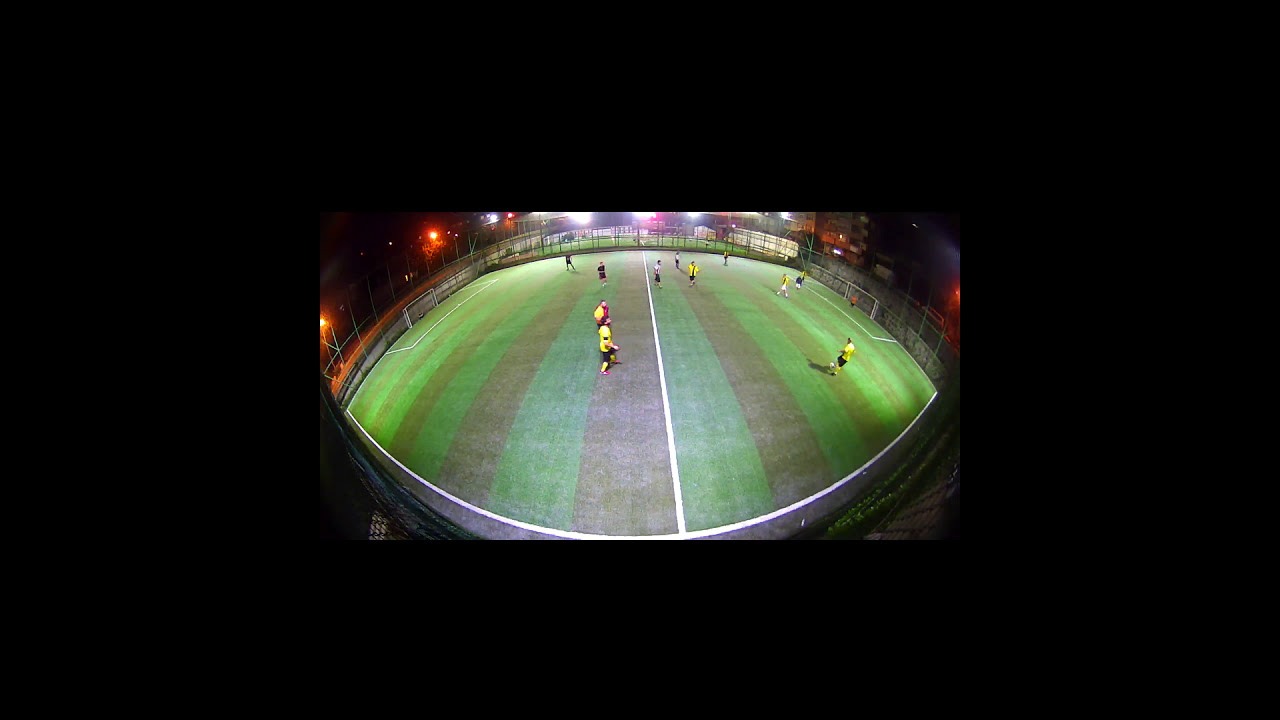In this captivating fisheye view of an outdoor soccer game at night, the image showcases a uniquely curved perspective due to the lens effect. The soccer field, which might be artificial turf given its finely cut, striped green pattern, is enclosed by a silver metal mesh fence for security. The field is oval-shaped, reminiscent of an eyeball, and is illuminated by a combination of amber and fluorescent lights, highlighting the surrounding dark area. Two goalposts mark the ends of the field, with a prominent white line running across the center and a white border around the field.

The match features players in distinct yellow jerseys—complemented with black shorts and yellow knee guards—with some players visible on both sides of the dividing line. While most players are dressed in yellow, one player stands out in a red shirt. The right side of the field has about six or seven players, while the left side has about three or four. The field appears to be pasted in the middle of a larger black rectangular area, making the vibrant scene pop against the dark backdrop. The combination of lighting and the night-time setting adds an intriguing glow to the dynamic soccer scene unfolding below.